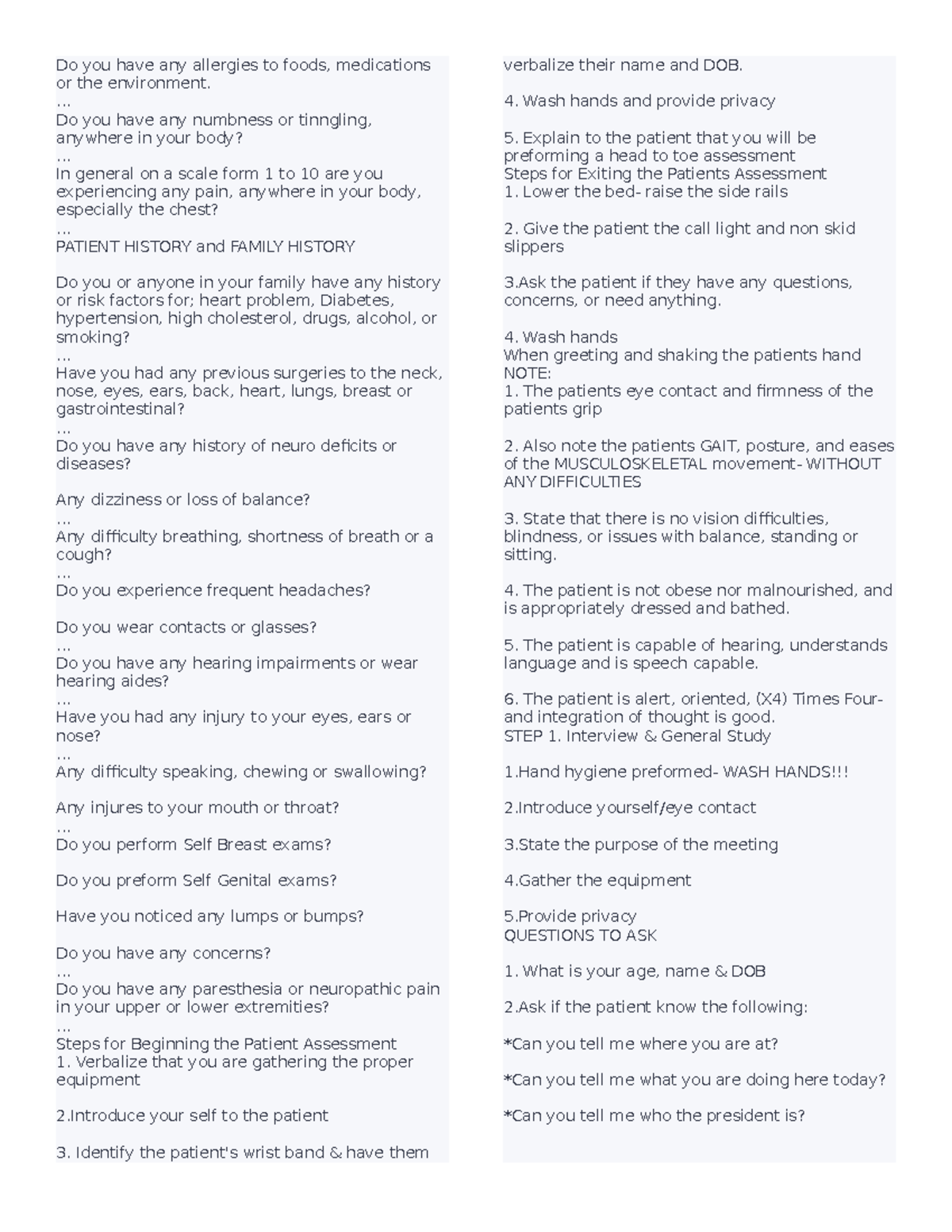The image consists of two adjacent panels set against a light gray background with charcoal gray text. 

The left panel features a series of medical questions aimed at assessing a patient's health conditions and risks. It begins with inquiries about any allergies related to food, medications, or the environment. This is followed by a question about numbness or tingling in any part of the body, where the word "tingling" is misspelled as "TINNGING". A pain assessment scale from 1 to 10 is included, with a focus on chest pain. Further, it delves into patient and family medical histories, asking about risk factors for heart problems, diabetes, hypertension, cholesterol levels, drug use, alcohol consumption, and smoking habits. The questionnaire also asks about any surgeries involving the neck, nose, eyes, ears, back, heart, lungs, breasts, or gastrointestinal tract. 

The right panel continues the line of questioning related to the patient assessment, numbering the steps sequentially. It begins with Step 1 and goes up to Step 3. The subsequent section picks up from Step 4 and continues to Step 5, then restarts from 1 and goes up to Step 6. Lastly, there's another set of four questions, labeled separately.

This detailed arrangement provides a comprehensive framework for assessing the patient's medical history and current health status.